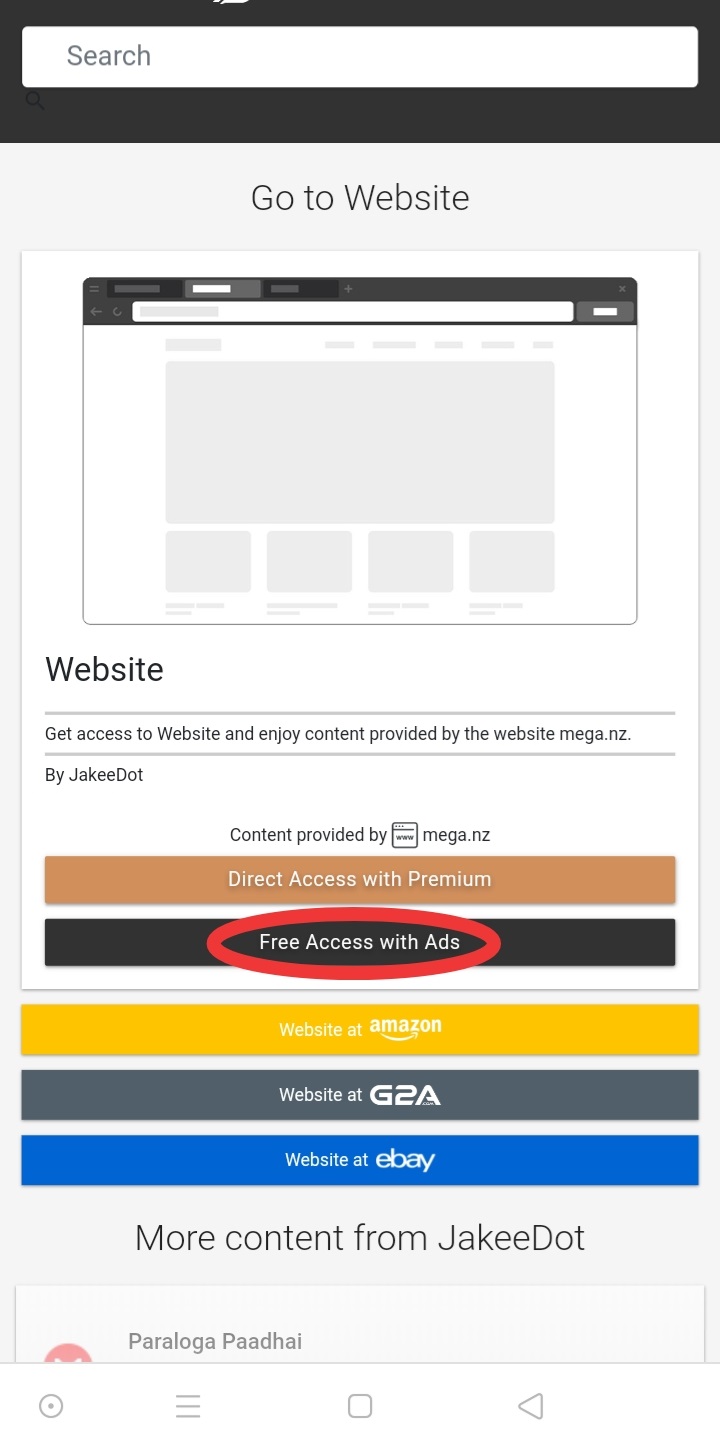The image displays a screenshot, set against a white background, featuring a structured interface. At the top, there is a black banner that houses a white search bar. Below the banner, grey text instructs users to "Go to website." 

Center-screen, a white box houses what appears to be an embedded screenshot of an additional layer of content. Prominently, "Website" is written in large black text above a horizontal grey line. Underneath, grey text reads, "Get access to website and enjoy content provided by the website Mega.nz by Jakey Dot." Centered within the white box, black text reiterates the source: "content provided by Mega.nz."

Towards the bottom of the interface, a series of buttons offer different actions. A camel-colored button labeled "Direct access with premium" is positioned centrally. Below this, a black button with white text, reading "Free access with ads," is circled in red to draw attention. Following this are three more buttons: a yellow one labeled "Website at Amazon," a grey one marked "G2A," and a blue button titled "Website at eBay."